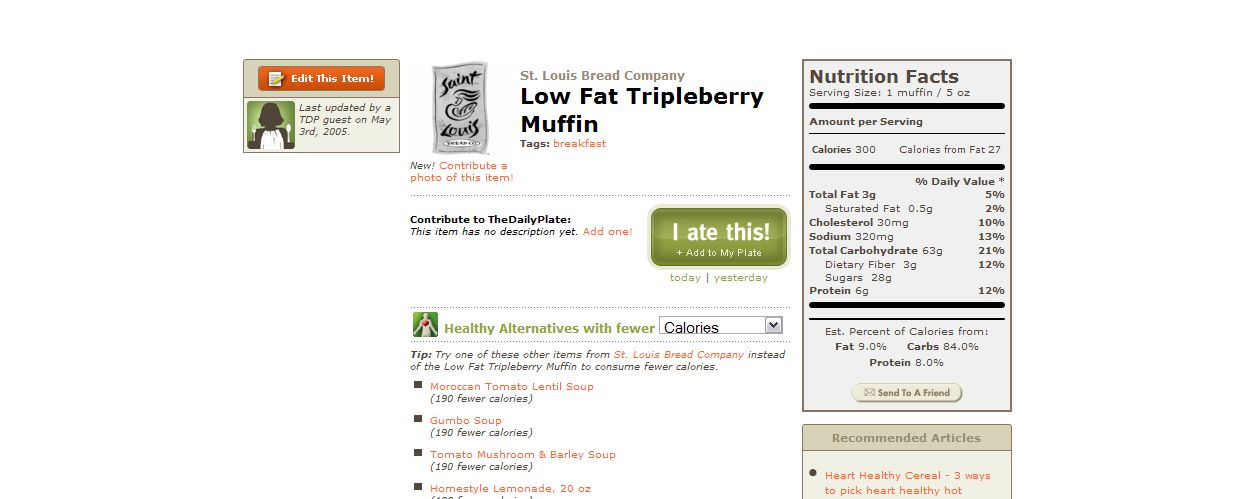The image depicts an old-style web page, likely a review or nutrition-tracking site, showcasing the low-fat triple berry muffin from St. Louis Bread Company. The layout is horizontal, indicating it's a screenshot from a computer. On the left side, the page features the St. Louis Bread Company logo at the top, followed by a prominent green button labeled "I ate this," encouraging user interaction. Beneath the button, the page offers guidance on healthy alternatives with fewer calories and lists other low-calorie items from the same company.

The central portion of the page highlights the product, the low-fat triple berry muffin, and mentions an update by a TDP guest on May 3, 2005. There is a prompt reading, "Contribute to The Daily Plate. This item has no description yet. Add one," suggesting users can add their reviews or descriptions. 

On the right side, the page displays a detailed nutrition facts table, although the small font makes it slightly difficult to read. Key nutritional information includes: one serving size equivalent to one 5-ounce muffin, containing 300 calories (27 from fat), 3 grams of total fat (5% daily value), 0.5 grams of saturated fat (2% daily value), 30mg of cholesterol (10% daily value), 320mg of sodium (13% daily value), 53 grams of total carbohydrates (21% daily value), 3 grams of dietary fiber (12% daily value), 28 grams of sugars, and 5 grams of protein (12% daily value).